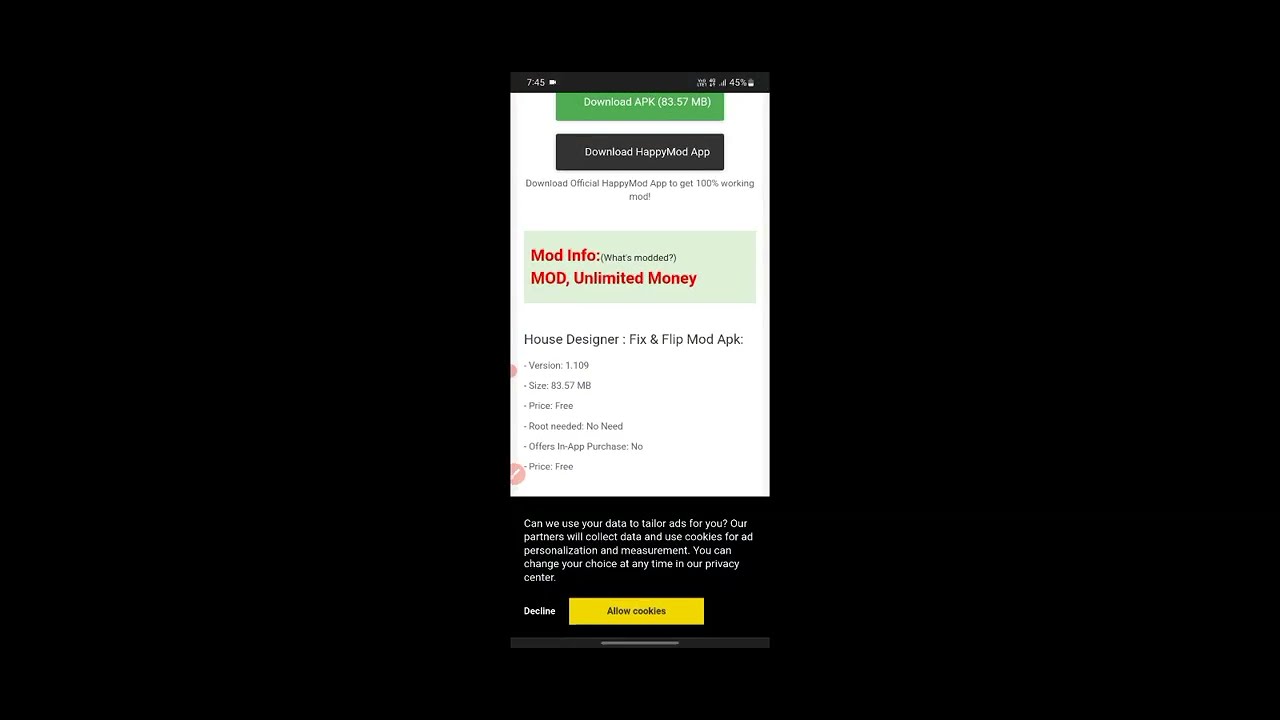This app screenshot on an Android phone screen features a black bar at the top displaying the time, temperature, battery level, and signal indicators. The main UI is a web browser window centered within a black background. At the top of the browser window, there is a large green button labeled "Download APK 83.7 MB," followed by a black button that reads "Download HappyMod App." Below these buttons, a descriptive text states, "Download official HappyMod app to get 100% working mod."

Further down, there's a light green box with red and black text that says, "Mod Info," followed by "What's Modded," and "Mod Unlimited Money." Below this, additional app details are listed, including "House Designer: Fix and Flip Mod APK Version 1.109," "Size: 83.57 MB," and "Price: Free." These details include bullet points clarifying that no root is needed and there are no in-app purchases.

Towards the bottom of the phone screen, there's additional white text on a black background, and at the very bottom, a yellow rectangle labeled "Allow Cookies" and above it, the white option to "Decline."